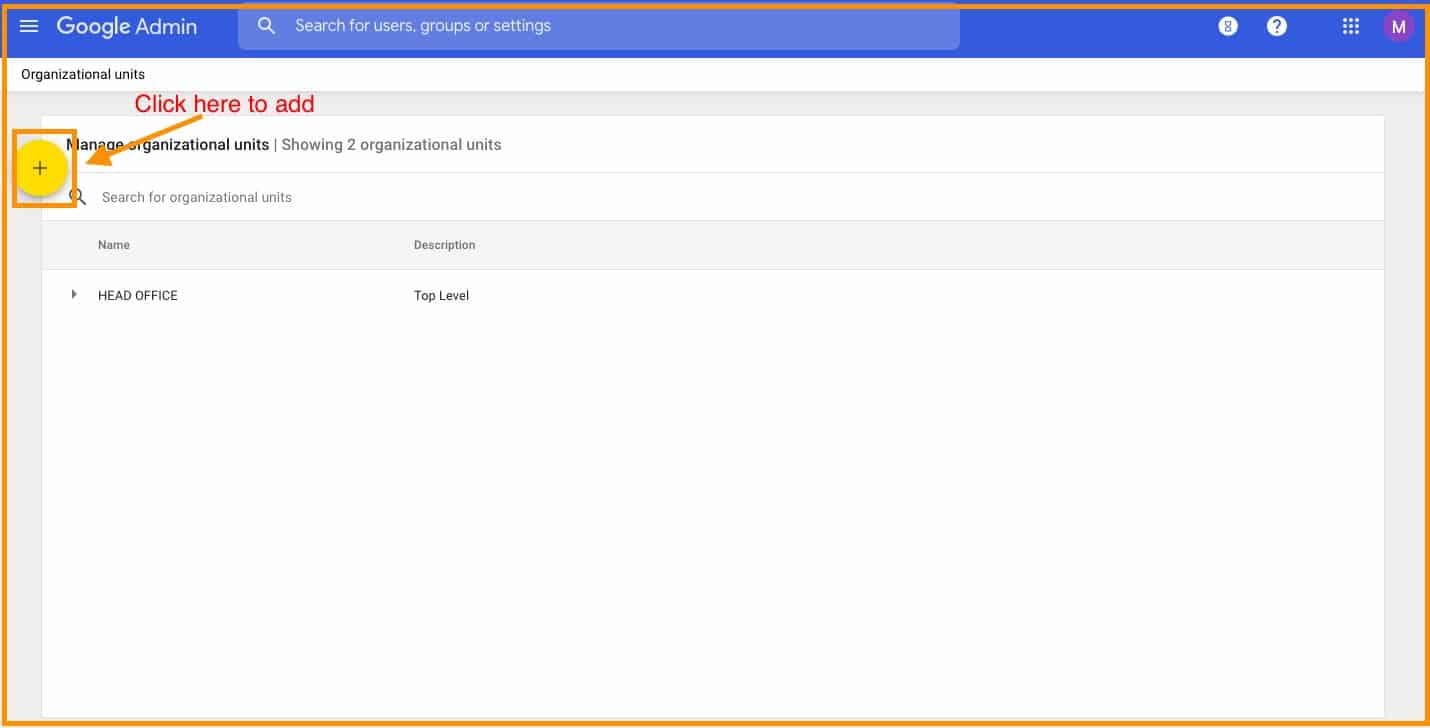The screenshot features a detailed interface from a desktop or laptop, likely from a Google Admin panel. At the top is a blue banner that extends across the screen. On the left side of this banner is a tab labeled "Google Admin" in white text next to a hamburger menu icon. Towards the center, there's a search bar with a light blue background and a magnifying glass icon. The text inside the search bar reads "Search for users, groups, or settings." On the far right of the banner, you'll find a set of icons: a Google icon, a question mark for help, a grid representing multiple Google apps, and an M icon, which likely represents the user.

Directly below the blue banner is a thin white banner with the text "Organizational units" on the far left. Beneath this banner is a section outlined in gray, containing organizational unit details. In the upper left corner of this section is a yellow circle with a plus sign, highlighted in orange, with an annotation and red arrow pointing to it. The annotation reads, "click here to add." 

This highlighted area partially obscures the underlying content but indicates actions related to adding organizational units. Below this highlighted section, there's a search bar for "search for organizational units," followed by columns named "Name" and "Description." The content within this table shows an entry labeled "Head Office" with an arrow icon suggesting it can be expanded to show more details. The description for "Head Office" is noted as "Top level." 

Additionally, almost the entire screenshot is accented with an orange bar, further emphasizing the highlighted sections and guide annotations.